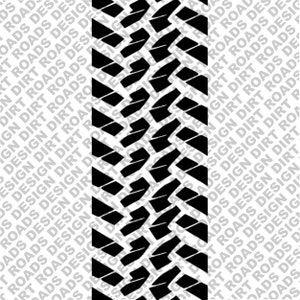The image depicts an abstract logo designed for a company likely involved in off-road activities such as dirt biking or off-road vehicling. The composition is square-shaped, utilizing a monochrome palette of black, white, and gray. The background is predominantly white with light gray capital letters diagonally repeating the phrases "Dirt Roads Design" from the lower left to the upper right corner. The repetition creates a textured overlay that covers the entire background. Positioned in the middle is a prominent black tire track imprint, which runs in a zigzag pattern from the top left to the bottom right of the image, occupying about one-third of the central area. The tire track is suggestive of the company's focus on dirt roads and design, emphasizing its connection to rugged, off-road environments.